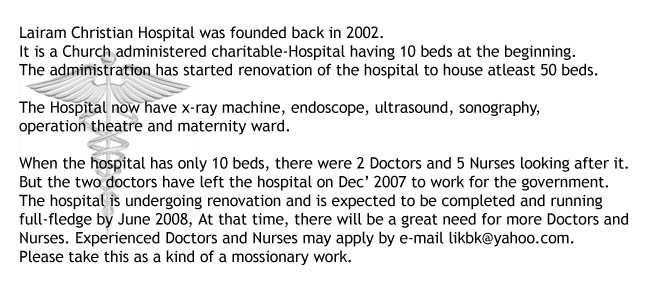The image features a black and white text paragraph that appears to be an advertisement in a publication, overlaid on a gray caduceus symbol representing the Medical Association. The text is aligned to the left, printed in black on a white background, and consists of several paragraphs. It details the history and current status of Lairam Christian Hospital, a church-administered charitable hospital founded in 2002. Initially, the hospital had 10 beds, staffed by two doctors and five nurses. As of December 2007, the two doctors left to work for the government. The hospital is currently undergoing renovations to expand to at least 50 beds, with an expected completion date of June 2008. The upgraded facility will include an x-ray machine, endoscope, ultrasound, sonography equipment, an operation theater, and a maternity ward. The notice calls for experienced doctors and nurses to apply by email at likbk@yahoo.com, emphasizing the mission-driven nature of the hospital's work.